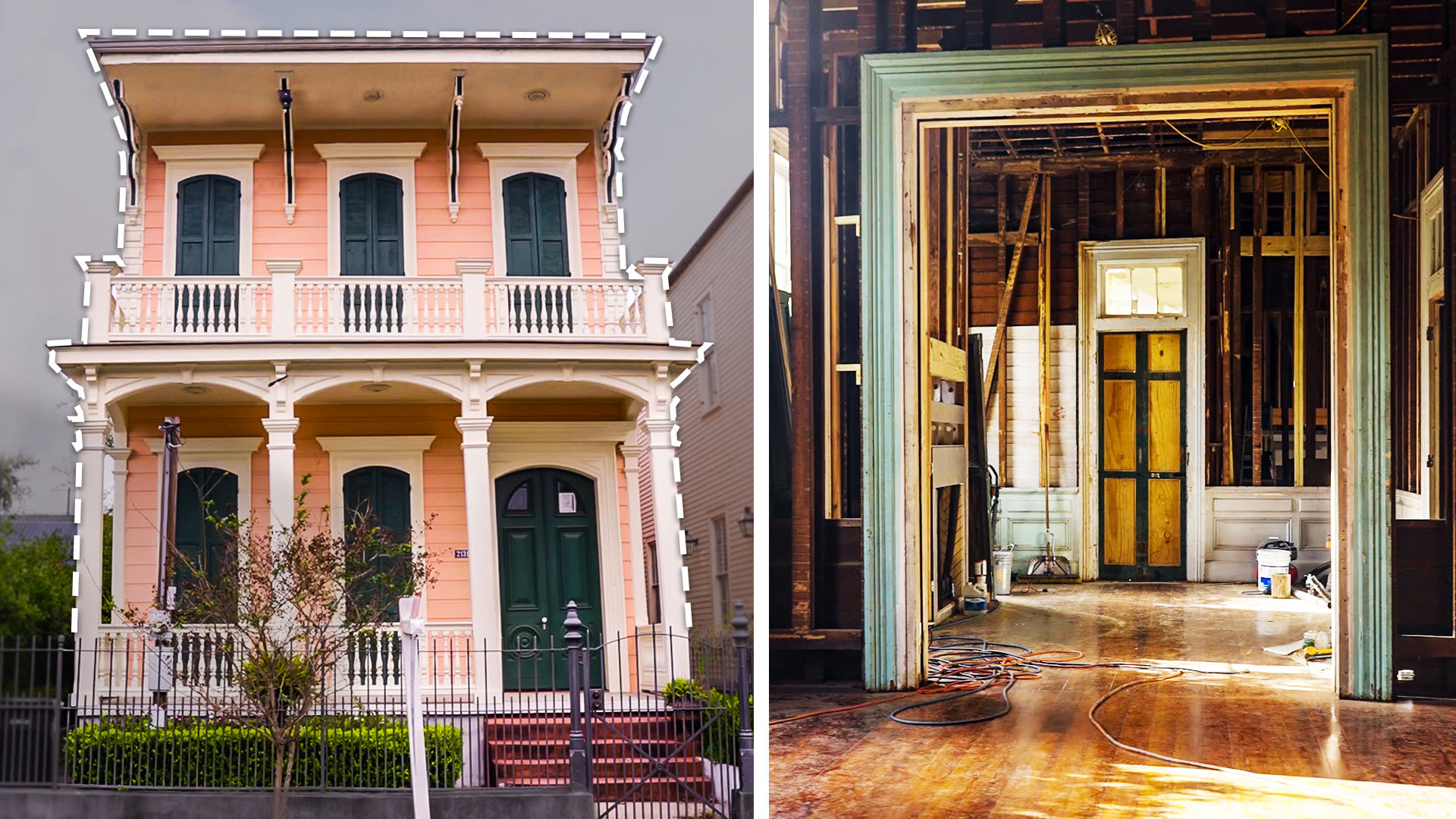The image is a horizontally aligned rectangular picture split into two vertical sections by a white line. The left section shows the front view of a two-story house painted pink with white borders around the windows and door. On the lower right, there's a dark green door, flanked by two windows to its left. The front porch has a white railing, similar to the one on the balcony above which stretches across three windows. The house is rectangular in shape with a wrought iron fence, about four to five feet high in front, and a row of bushes along the left side. The scene appears on a cloudy day with a gray sky overhead.

The right section reveals the interior of this house, which is under renovation. The room features wood tile flooring, an arched or framed-out doorway without a door, scattered extension cords, paint cans, and an assortment of tools on the floor. The walls and ceiling remain unfinished, showing exposed studs. The entire setting is brightly lit and clearly visible.